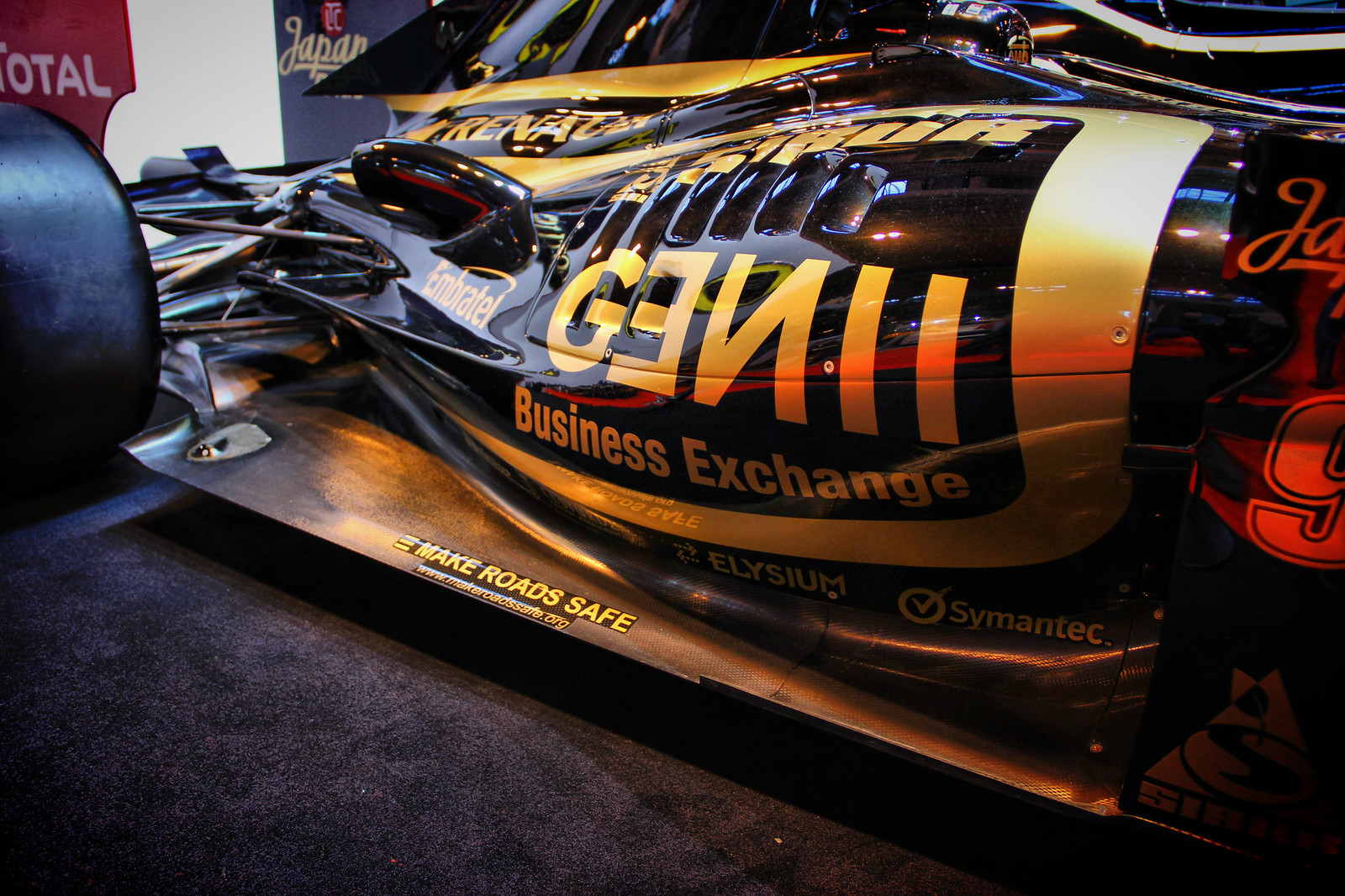This close-up photograph, taken indoors with low showroom lighting, captures what appears to be a sleek and shiny black race car adorned with gold trim and set against a black pedestal. The race car, featuring big, fat black wheels, has a distinctive and elegant appearance. Central to the image is an oval-shaped black and gold object, which extends outwards into a tail-like structure. The object is framed with gold paint and prominently displays the text "GENii Business Exchange" in gold font, albeit with some letters appearing reversed.

At the bottom of the object, there's a gold-colored footplate or skid plate with a yellow and black sticker that reads "Make Roads Safe." Above this, the car's dark door with a reddish tint, likely caused by the lighting, showcases cursive writing that begins with "J A," indicating the word "Japan." A silver or metallic area below the business exchange lettering further reiterates the "Make Roads Safe" message. On the background wall, visible behind the race car, are posters with distinct sections: a red stripe with "Total" in white, a white stripe, and a black stripe with "Japan" in gold cursive, echoing the text on the vehicle. The overall setting includes a dark gray carpet on the bottom left corner, adding to the upscale showroom ambiance.